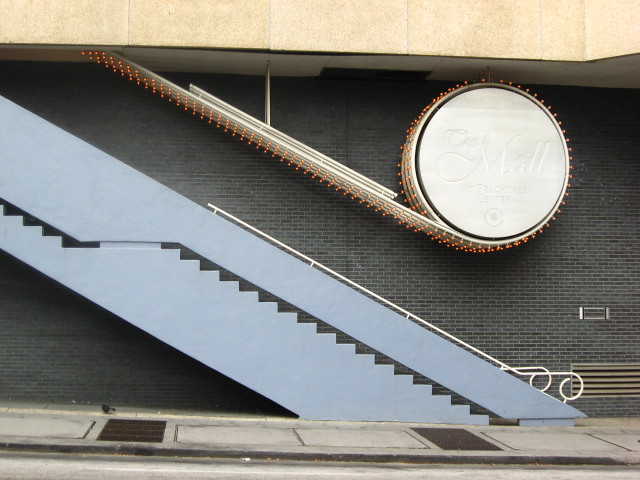This detailed photograph captures an exterior view of part of a building, prominently featuring a light gray stone staircase descending diagonally from the upper left to the bottom right of the image. Beside this staircase, which is equipped with a white handrail that elegantly swirls at the end like a cane, there is another staircase likely functioning as an escalator. Both staircases converge near a sidewalk at the base.

Above and to the right of this stone staircase, an ornate circular light sign prominently displays the words "The Mall." The sign, reminiscent of an unraveling roll of tape, is detailed with tiny, red light bulbs that create an intricate pattern around its edge and continue in a line along the contour of the stairway. This entire scene is set against the backdrop of a gray brick wall, adding a textured contrast to the smooth, illuminated sign and structural elements of the staircases.